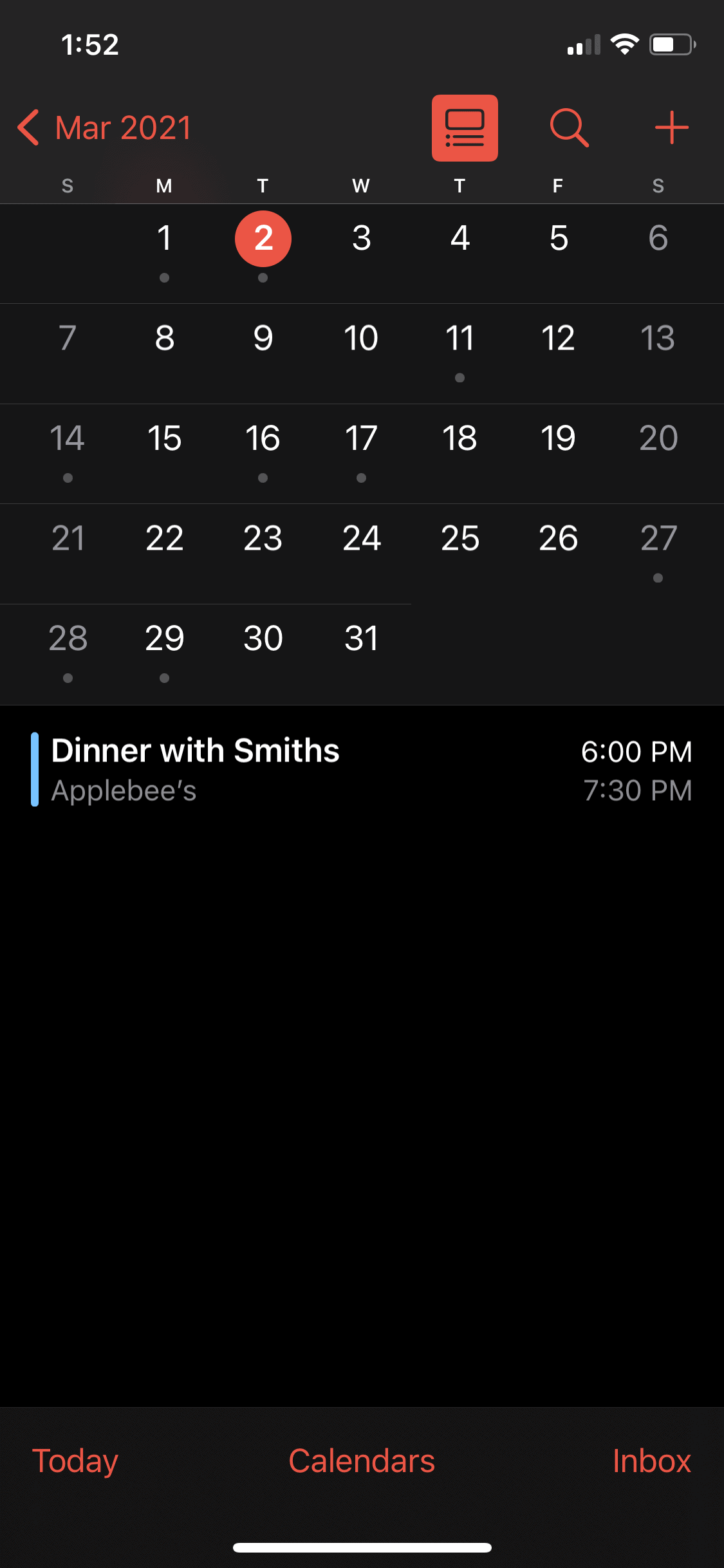This is a detailed screenshot of a smartphone interface displayed against a black background. In the top left corner, the time reads 1:52. The top right corner indicates a partially filled signal bar at 2 out of 4, a full Wi-Fi signal, and a battery life at approximately 50%. Below the time, the date "March 21" is displayed in red, accompanied by a leftward arrow. To the right of the date is a blank space, followed by a square icon featuring another square and red lines, a red magnifying search icon, and a red plus icon.

The main portion of the screenshot features a calendar view. The days of the week are abbreviated, with Sunday (S) on the far left and Saturday (S) on the far right. Monday is marked as the 1st, Tuesday as the 2nd (circled in red), and the 31st falls on a Wednesday. Below the calendar, there is an event titled "Dinner with Smiths" at "Applebees." A blue vertical line is positioned to the left of these details. To the right, the event time is initially listed as 6:00 pm, followed by a subsequent time of 7:30 pm.

The bottom section of the screenshot is again a black background, featuring navigation options. The options, written in red, are "Today" on the far left, "Calendar" in the center, and "Inbox" on the far right.